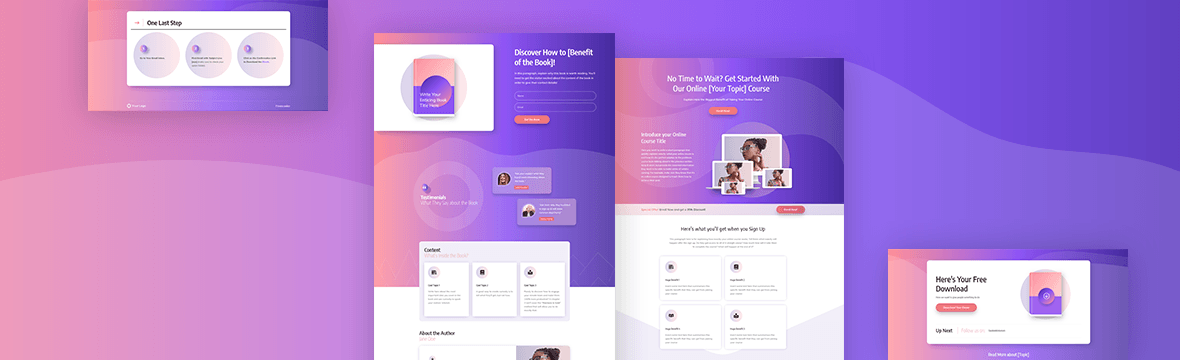The image is a vibrant, visually appealing advertisement page with a predominantly purple-lilac and pinkish color scheme, featuring wavy patterns throughout. 

In the top-left corner, bold text reads "Get One Last Stop." Below that, another headline states, "Discover How to Benefit from the Book." Towards the bottom of the page, several additional pieces of text are displayed, contributing to the overall aesthetic and informative design.

One of the prominent messages is, "No Time to Wait. Get started with our online 'Your Topic' course," encouraging engagement. The final piece of text offers a call to action: "Here's Your Free Download," accompanied by a download button for an application, suggesting that this is indeed an advertisement for an app.

The design not only catches the eye with its lively colors and dynamic layout but also effectively communicates multiple compelling messages to the viewer.